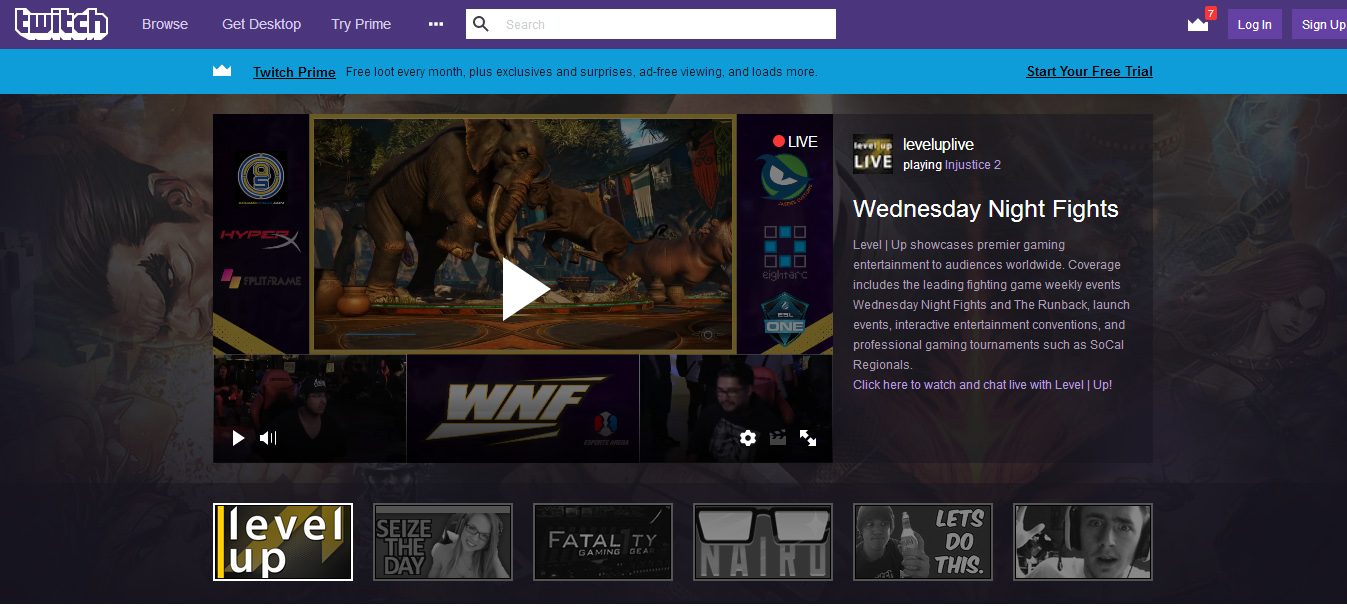This horizontal screenshot captures the Twitch website interface in great detail. At the top-left corner, the familiar Twitch logo and name are prominently displayed on a purple banner, which spans the width of the screen. Adjacent to the logo, the navigation options "Browse," "Get Desktop," and "Try Prime" are clearly visible. Centrally placed within the banner is a search box for easy access, while the right-hand side features login and signup buttons for user convenience.

Beneath the primary banner, there's a blue secondary banner highlighting Twitch Prime benefits. The text reads "Twitch Prime" underlined, followed by promotional points such as "Free Loot Every Month, Plus Exclusives and Surprises," "Ad-Free Viewing," and additional perks. A "Start Your Free Trial" link concludes this informative section.

Dominating the center of the screen is a large game thumbnail for "Wednesday Night Fights," showing an arena battle scene with elephants and other animals. A play button, depicted as a right-facing white arrow, is superimposed on the image, indicating that it is a live stream. The live status is further emphasized by a red dot and the word "LIVE."

A translucent gray overlay partially obscures the background to ensure focus remains on the game's content, while a character of a man is subtly visible behind this pop-up box on the left. At the bottom of the screenshot, six game icons are arranged in a row, with the leftmost icon marked "Level Up." This icon features a distinctive yellow strip and is highlighted in white, suggesting it is currently selected or of special importance.